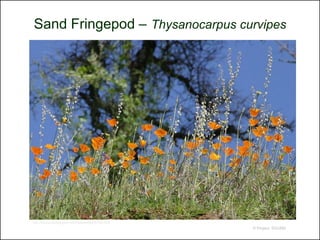This photograph, bordered in black with a white background, appears to be a detailed educational image likely from a textbook or guidebook. At the top of the image in black type, the text reads "Sand Fringe Pod – Thysanocarpus curvipes," indicating both the common and scientific names of the flowers depicted. Below this caption, the image showcases a vibrant field of flowers, predominantly golden and orange in color, reminiscent of California poppies, standing tall amidst green vegetation and some smaller white flowers interspersed among them. The scene is set against a backdrop featuring a slightly blurry green tree and a clear blue sky, adding depth and natural context to the composition. The bright orange flowers, which bloom individually and stand out vividly against the surrounding shrubbery, contrast beautifully with the diverse flora, capturing a picturesque moment of nature's splendor.